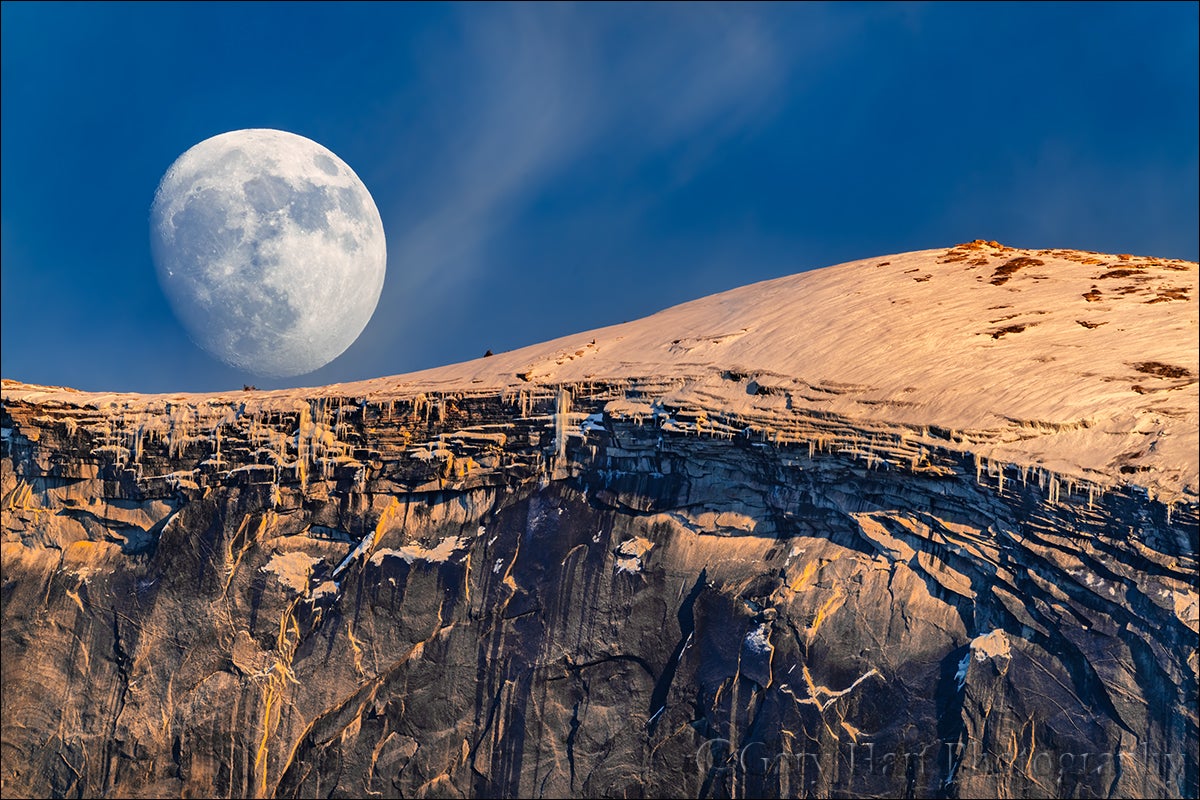This professionally taken, highly detailed image showcases a stunning outdoor scene that almost appears digitally altered. The focal point is a granitic cliff with hues of gray, tan, and black, extending up towards the right side. Striations and signs of erosion are evident along the cliff face, which descends steeply to the bottom of the picture. Atop the cliff, a sandy terrain with yellow-brown brush adds contrast, indicative of a desert environment. The most striking feature is the immense moon on the left side of the image, so large and detailed that its craters are clearly visible, giving the illusion that the moon is exceptionally close. The bright blue sky accentuates the scene, providing a vivid backdrop to this captivating juxtaposition of natural elements.